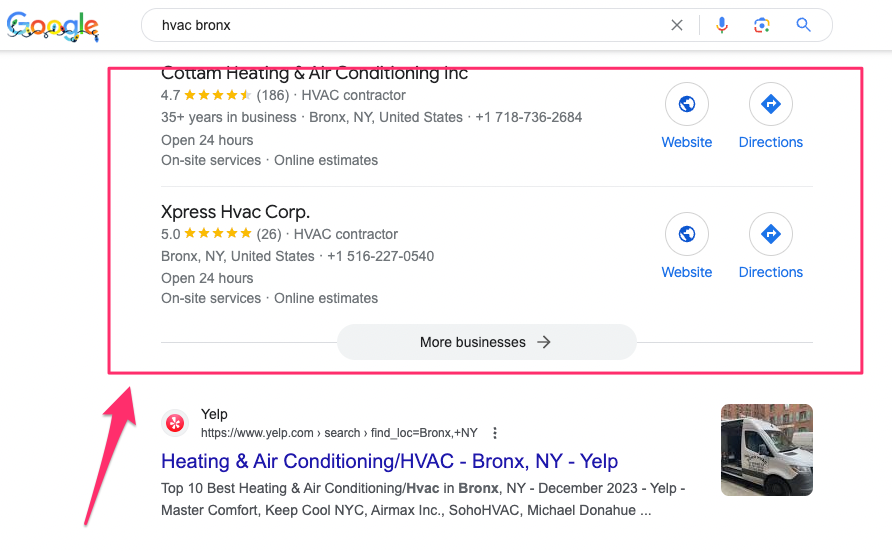A detailed screenshot shows a Google search results page for the query "HVAC Bronx." The search term is visible in the search bar at the top. A red rectangle highlights the first two listings in the search results. The first listing is for "Cotham Heating and Air Conditioning, Incorporated," which has a rating of 4.7 stars based on 186 reviews. The company is identified as an HVAC contractor with 25 years in business, located in Bronx, New York, USA. Their contact number is 718-736-2684, and they offer 24-hour operation, on-site services, and online estimates.

The second highlighted listing is for "Express HVAC Corp," which boasts a 5-star rating from 26 reviews. This company is also an HVAC contractor based in Bronx, New York, USA, with the contact number 516-227-0540. They similarly offer 24-hour services, on-site services, and online estimates.

Below the red rectangle, there is another listing from Yelp with the URL "www.yelp.com." The summary mentions a search feature to find HVAC services in Bronx, New York, and references the top 10 best-selling heating and air conditioning services in the Bronx as of December 2023.